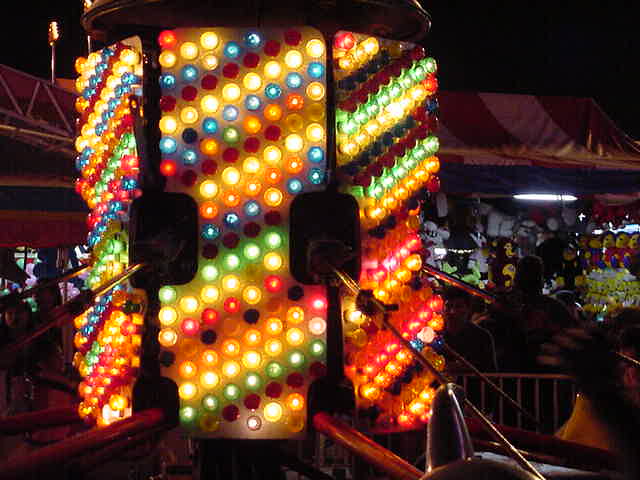This nighttime photograph captures a bustling carnival scene, with the central focus being a large, cylindrical column adorned with an array of colorful light bulbs. The column, possibly part of a carnival ride, features panels of lights arranged in diagonal patterns, incorporating vibrant hues of red, green, blue, yellow, and gold. Illuminating the dark surroundings, these lights create a striking visual effect. Surrounding the column are four sharp beams or poles pointed toward it, adding to the dynamic scene. In the background, a booth filled with stuffed animals is visible, further emphasizing the lively and festive atmosphere of the fairground.